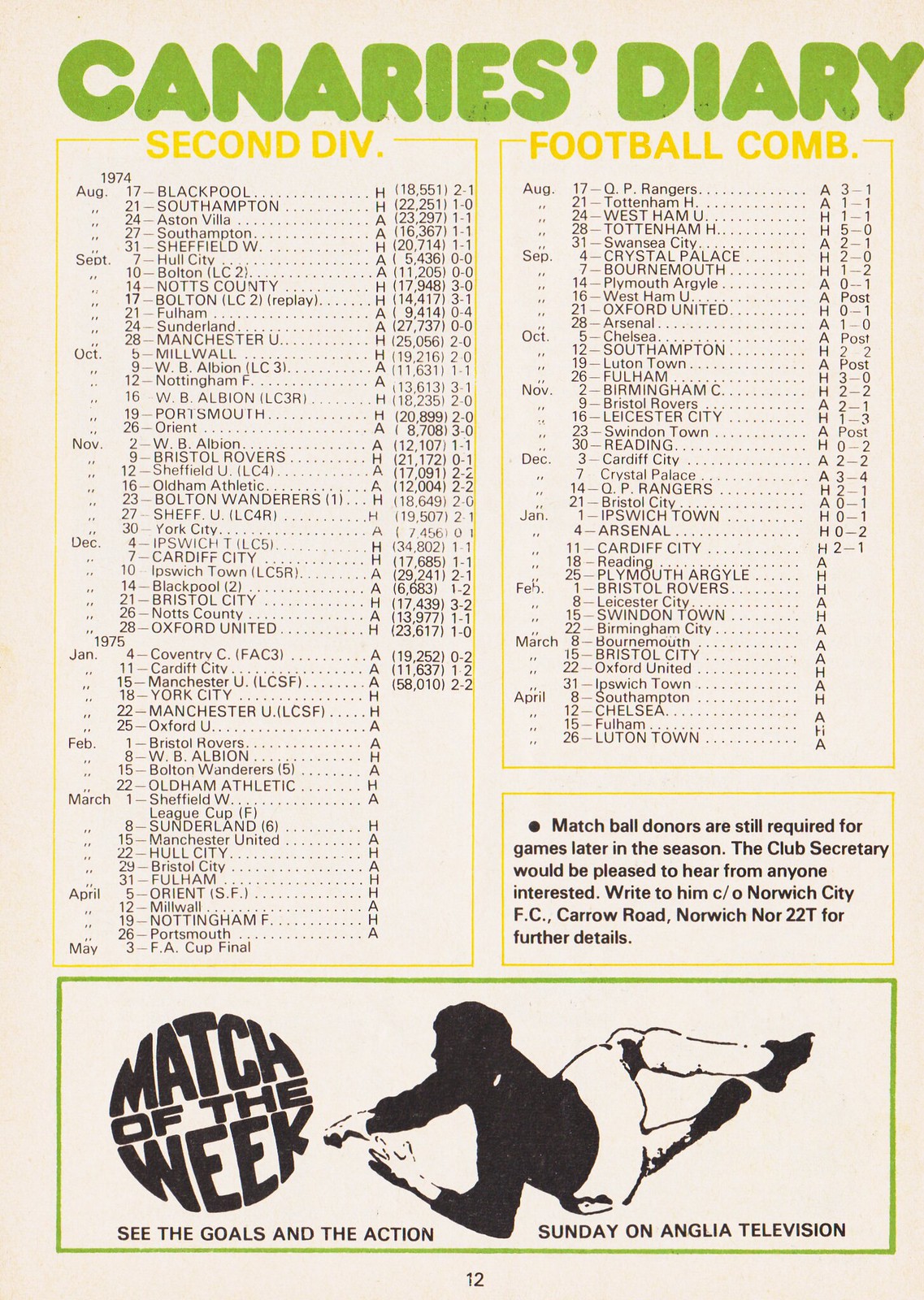In the image, we see a vintage football program titled "Cannery's Diary" at the top in green text. The central piece, set against a tan background, lists matches for the 2nd Division Football, spanning dates from August 1974 through May 3rd. On the left side, there's a yellow text section labeled "Second Div," and on the right side, it reads "Football C-O-M-B," which might signify a combination or abbreviation of terms.

At the bottom of the program, there is an illustration of a football player attempting to catch a ball, with the ball formed by the words "Match of the Week" in black text inside a green box. Beneath this, the text reads, "See the Goals and the Action, Sunday on Anglia Television." Additionally, above this illustration, a paragraph indicates, "Match ball donors are still required for games later in the season. The club secretary would be pleased to hear from anyone interested. Write to him, C-O-M-B." The colors throughout the program include tan, green, yellow, and black, and its overall layout suggests it could be a page from a sports magazine or a promotional poster.